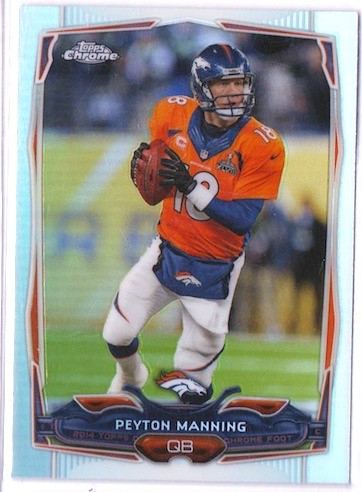This image features a limited edition, holographic football card encased in a clear plastic protector. The card showcases famed quarterback Peyton Manning in his 2014 Denver Broncos uniform. Manning is depicted mid-action, holding a brown football while wearing black gloves, white wristbands, a blue undershirt, an orange and blue jersey with the number 18, and a blue and orange helmet. His white pants are complemented by a blue and black fanny pack adorned with the iconic white and orange Broncos head logo. The top left corner of the card displays "Topps Chrome" in white letters on a silver background, highlighting its special edition status. At the bottom, his name "Peyton Manning," his position "QB," and the year "2014" are clearly printed in white letters on a blue background. The card's border is a mix of blue, orange, and gray tones that accentuate its metallic and holographic finish. Behind Manning, the green football field with white stripes and out-of-focus audience members add to the dynamic scene.